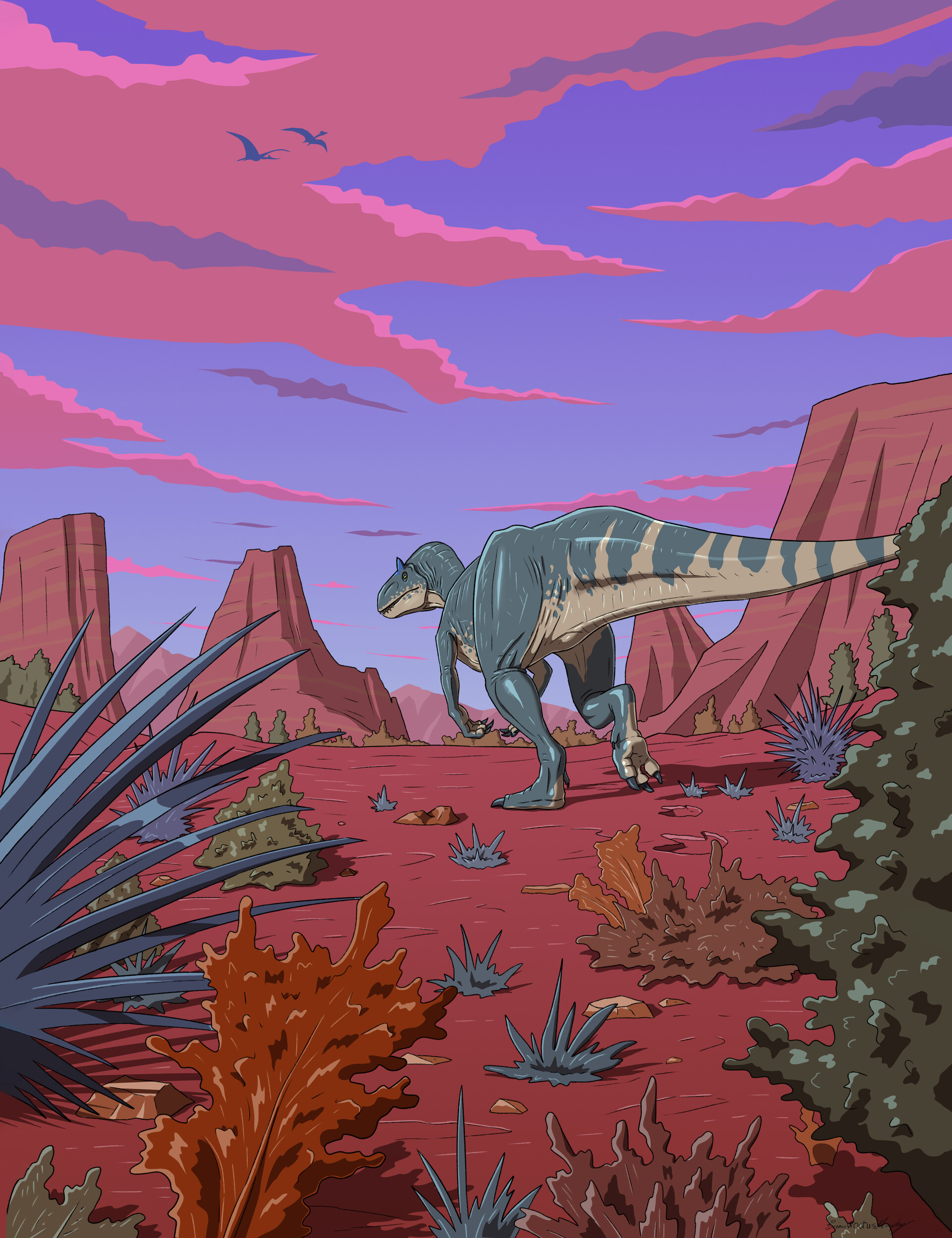An animated illustration depicts a prehistoric outdoor scene with a dinosaur, likely a Tyrannosaurus rex, at its center. The dinosaur is facing away from the viewer and appears to be walking to the left. It is characterized by its pale green and beige coloring, with a lighter yellow underbelly and underside. Its tail has a distinctive pattern that alternates between green and white. The T-Rex's right foot is lifted, while its left foot is firmly planted on the ground. The scene is set within a desert-like plateau area featuring pinkish and light red mountain bluffs in the background. 

The foreground showcases a variety of cartoonish desert plants and bushes, including a dark green pine tree in the bottom right corner, along with green, orange, blue, and brown bushes scattered across the red dirt ground. The sky overhead is a gradient of dark blue to purple, becoming lighter near the horizon, and is filled with pinkish-red clouds. Two pterodactyls can be seen in the distance in the top left part of the sky.